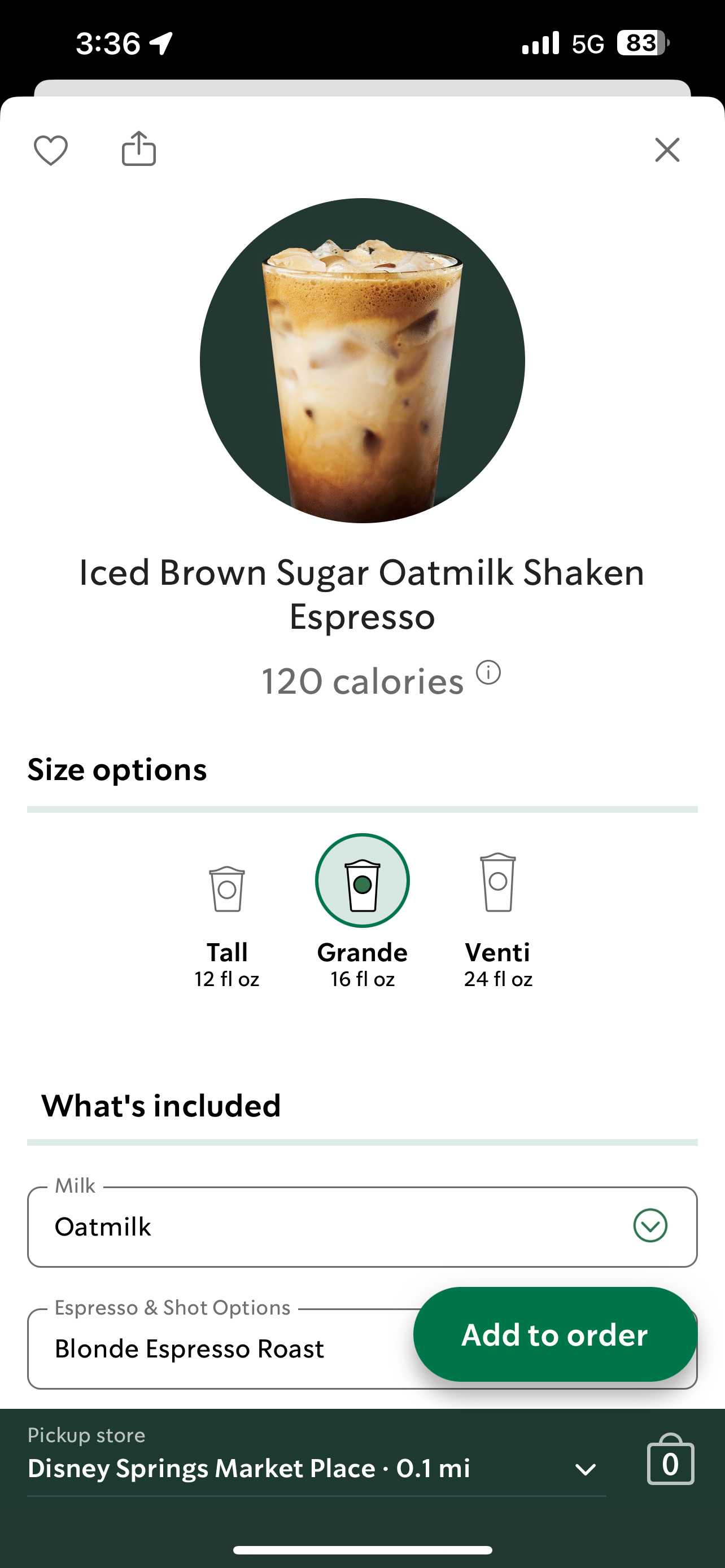At the top of the image, there's a black bar featuring the number "336" accompanied by a paper airplane icon. Adjacent to this, on the right-hand side, four horizontal lines of increasing length are shown, indicating a strong mobile signal. The display also shows "5G" connectivity and a mostly filled battery icon with 83% remaining. 

The main section below is predominantly white. To the left, a gray-outlined heart icon is visible, and next to it is a gray-outlined rectangle with an upward-pointing arrow, followed by a gray 'X' icon on the far right.

At the center, a green circle encloses an image resembling a coffee drink, specifically an iced beverage labeled "Ice, Brown Sugar, Oatmilk, Shaken Espresso." Beneath this, the calorie content is stated: "120 calories."

Further down, on the left, the text "Size Options" is displayed above a green line. This line leads to illustrations of different cup sizes: the smallest labeled "Tall, 12 FL OZ," followed by "Grande, 16 FL OZ" within a green-circled cup, and finally "Venti, 24 FL OZ" outlined.

"What's included" is presented in black text above another green line. Below, there are sections specifying customizable options starting with "Milk," which has a rectangular label with "Oatmilk" on it. A green circle with a check mark confirms the selection.

Next, "Espresso and Shot Options" is detailed, featuring the choice "Blonde Espresso Roast." An adjacent green button with bulging sides states "Add to Order."

Towards the bottom, a dark green rectangle with "Pick Up Store" directs users to "Disney Springs Marketplace, 0.1 MI." An arrow points downward to a shopping bag icon with an 'O' in it, completing the layout with a thin white line at the image's base.